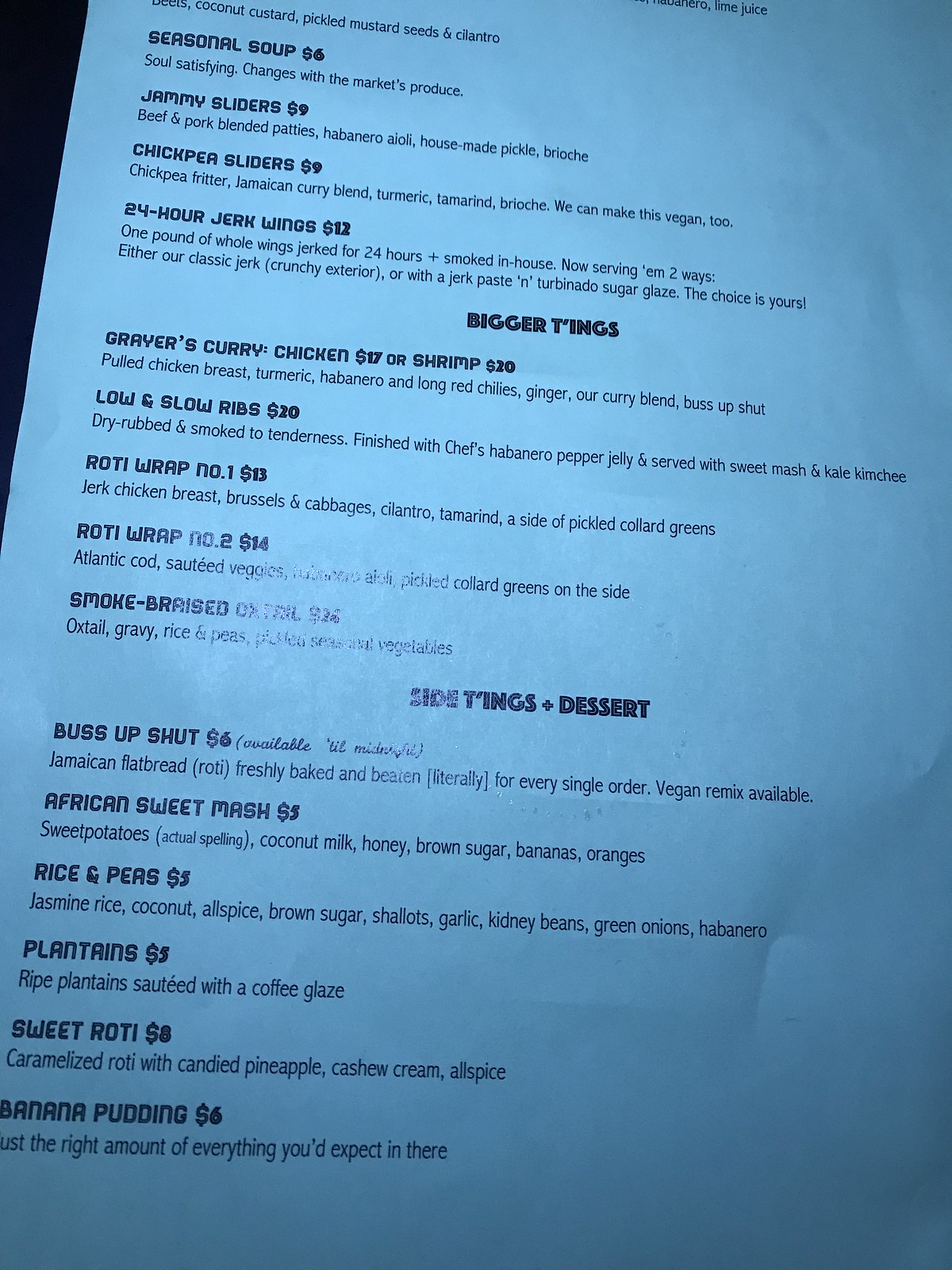Close-up of a Menu on Light Blue Paper:
 
The photograph showcases a close-up view of a menu printed on light blue paper. Due to the quality of the camera, the true color may be slightly distorted. The top of the menu isn't visible, but the detailed text includes a variety of mouthwatering dishes and beverages.

**Starters:**
- **Lime Juice**
- **Coconut Custard**
- **Pickled Mustard Seeds**
- **Cilantro**

**Seasonal Soup**:
- **$6**: Soul-satisfying soup that changes with the market’s produce.

**Jammy Sliders**:
- **$9**: Beef and pork blended patties with house-made pickles and habanero aioli on brioche.

**Chickpea Sliders**:
- **$9**: Chickpea fritter spiced with Jamaican curry blend, turmeric, and tamarind, served on brioche. Vegan option available.

**24 Hour Jerk Wings**:
- **$12**: One pound of whole wings marinated and jerked for 24 hours, smoked in-house, served either as classic jerk with a crunchy exterior or jerk with jerk paste and turbinado sugar glaze.

**Bigger Tings:**
- **Greyer's Curry Chicken**: **$17** or **Shrimp**: **$20**: Pulled chicken breast with turmeric, habanero, long red chilies, ginger, and house curry blend, served with Bus up shut.
- **Low and Slow Ribs**:
  - **$20**: Dry rubbed and smoked to tenderness, finished with chef’s habanero pepper jelly, served with sweet mash and kale kimchi.
- **Roti Wrap Number One**:
  - **$13**: Jerk chicken breast with Brussels, cabbage, cilantro, tamarind, and a side of pickled collard greens.
- **Roti Wrap Number Two**:
  - **$14**: Atlantic cod with sautéed veggies and a side of pickled collard greens.
- **Smoked Braised Oxtail**:
  - **$24**: Oxtail served with gravy, rice and peas, and pickled seasonal vegetables.

**Side Tings Plus Dessert:**
- **Bus up shut**:
  - **$6**: Jamaican flatbread roti, freshly baked and beaten for each order. Vegan remix available.
- **African Sweet Mash**:
  - **$5**: Sweet potatoes blended with coconut milk, honey, brown sugar, bananas, and oranges.
- **Rice and Peas**:
  - **$5**: Jamaican rice cooked with coconut, allspice, brown sugar, shallots, garlic, kidney beans, green onions, and habanero.
- **Plantains**:
  - **$5**: Ripe plantains sautéed with a coffee glaze.
- **Sweet Roti**:
  - **$8**: Caramelized roti topped with candied pineapple, cashew cream, and allspice.
- **Banana Pudding**:
  - **$6**: A perfectly balanced dessert with all the expected traditional flavors.

The menu offers a rich variety of Caribbean-inspired dishes, providing both bold flavors and comforting choices for a diverse palate.